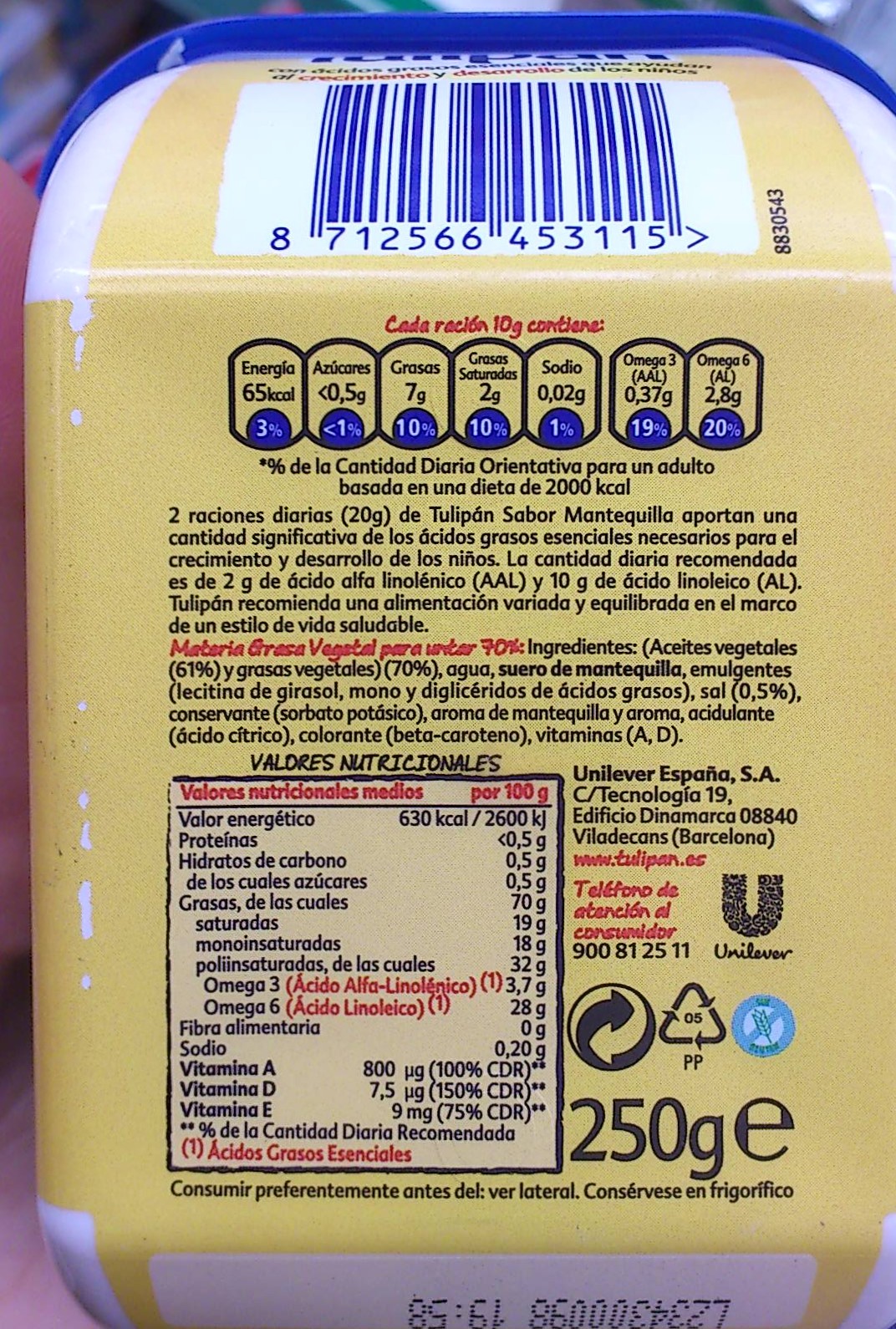The image captures the back of a yellow food package with a blue trim and white edges, positioned inside a blue pail. The label, written primarily in a foreign language—likely Spanish—contains detailed nutritional information, including vitamins A, D, and E, and mentions ingredients such as various vegetables and emulsifiers. At the bottom right corner, the weight is marked as 250G, while a Best Buy date is noted at the bottom. The top of the package features a barcode. In the blurred background, other food packages are faintly visible. The package appears firm, suggesting it might be tightly packed or within a plastic container.